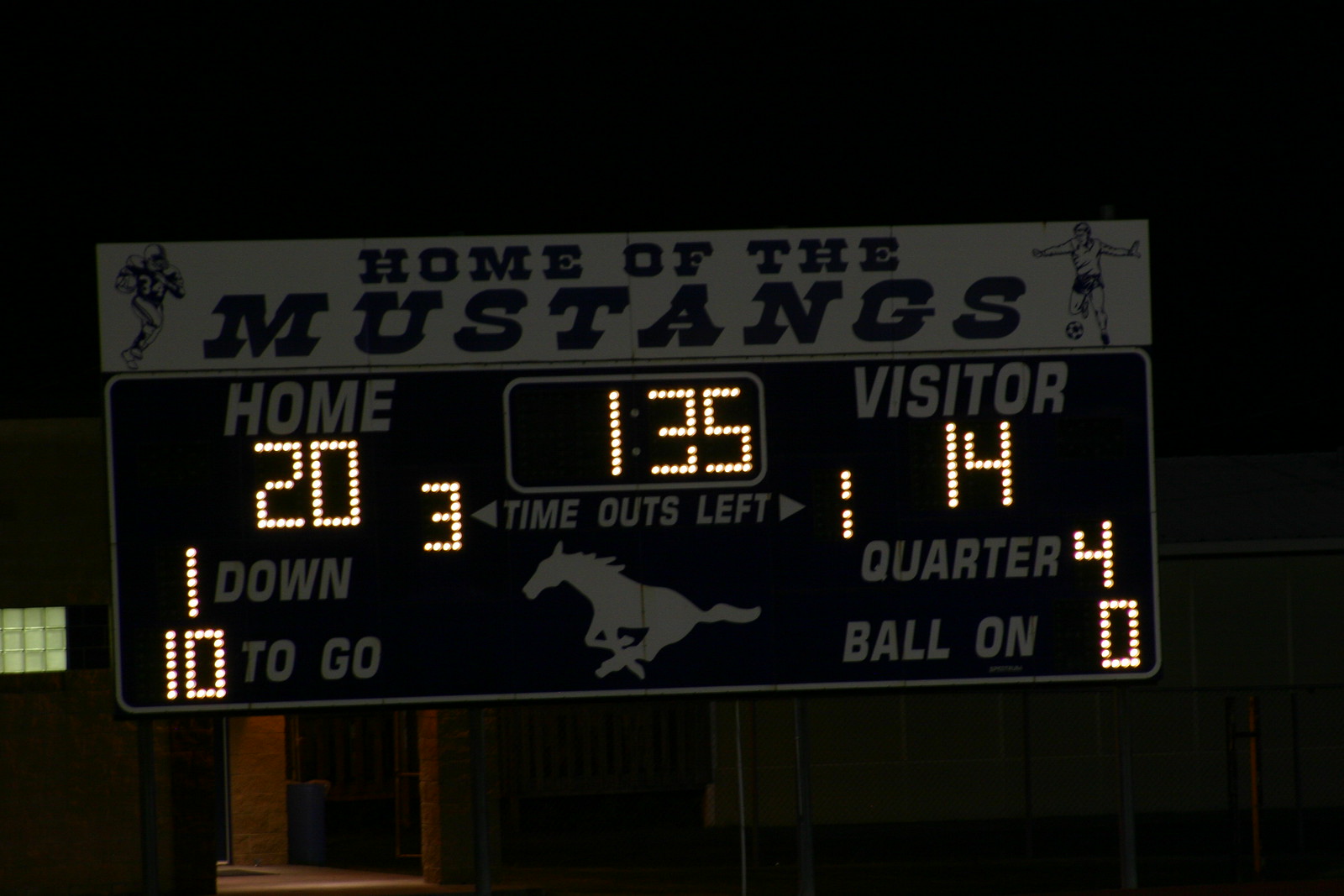This nighttime photograph captures an outdoor football stadium scoreboard prominently displaying the phrase "HOME OF THE MUSTANGS" in italicized, all-uppercase white letters. Set against a dark backdrop, the black scoreboard is illuminated by lightbulbs, clearly showcasing the current score and game details: Home team leads with 20 points, while the Visitors have 14 points. The scoreboard indicates there is 1 minute and 35 seconds left in the fourth quarter, with the ball on the zero-yard line and a 10-yard advance needed for the first down. The Home team has 3 timeouts remaining, whereas the Visitors have 1. Accompanying these details are multiple graphics, including a horse logo representing the Mustangs and two athlete illustrations—one of a runner wearing number 34 and another of a soccer player positioned on the far right. The scene is devoid of spectators, maintaining a focus on the illuminated scoreboard amidst the surrounding darkness.